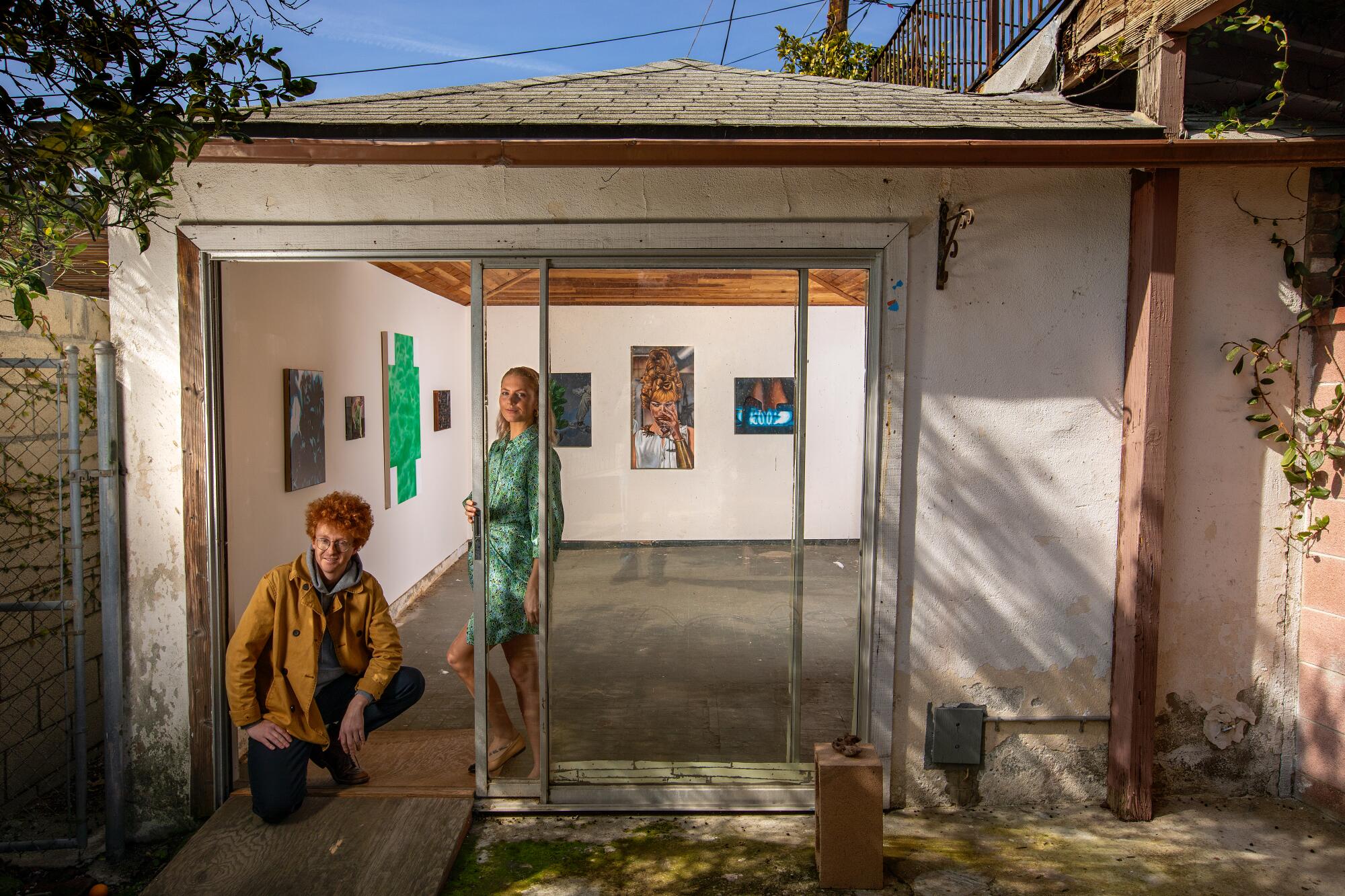This photograph captures an art gallery setup in what appears to be a converted, dilapidated garage or storage area. The building has white stucco walls and a sliding glass door at the entrance, above which blue skies with thin clouds and power lines are visible. A wooden ramp leads up to the entrance, making it accessible for hand carts. 

Inside the gallery, the white walls are adorned with five paintings and drawings; one prominent piece features a green cross shape, and another depicts a figure with a hat. The wooden floor appears unfinished, giving the space an under-construction feel. 

In the image, a young man, likely in his 20s, is kneeling near the entrance, wearing a yellow jacket, dark pants, a red earring, and glasses. Beside him stands a woman with wide brown hair, dressed in a short green and white dress. Her left leg is bent forward while her right leg remains straight. 

To the left of the building is part of a chain-link fence, and an electrical box is visible. The foreground features a brown, block-shaped object and some gray elements on the building’s wall. Ivy climbs up a brick wall on the right side. The surrounding area includes spotty grass, soil, green tree limbs, and bushes, adding a touch of nature to this artistic setting.